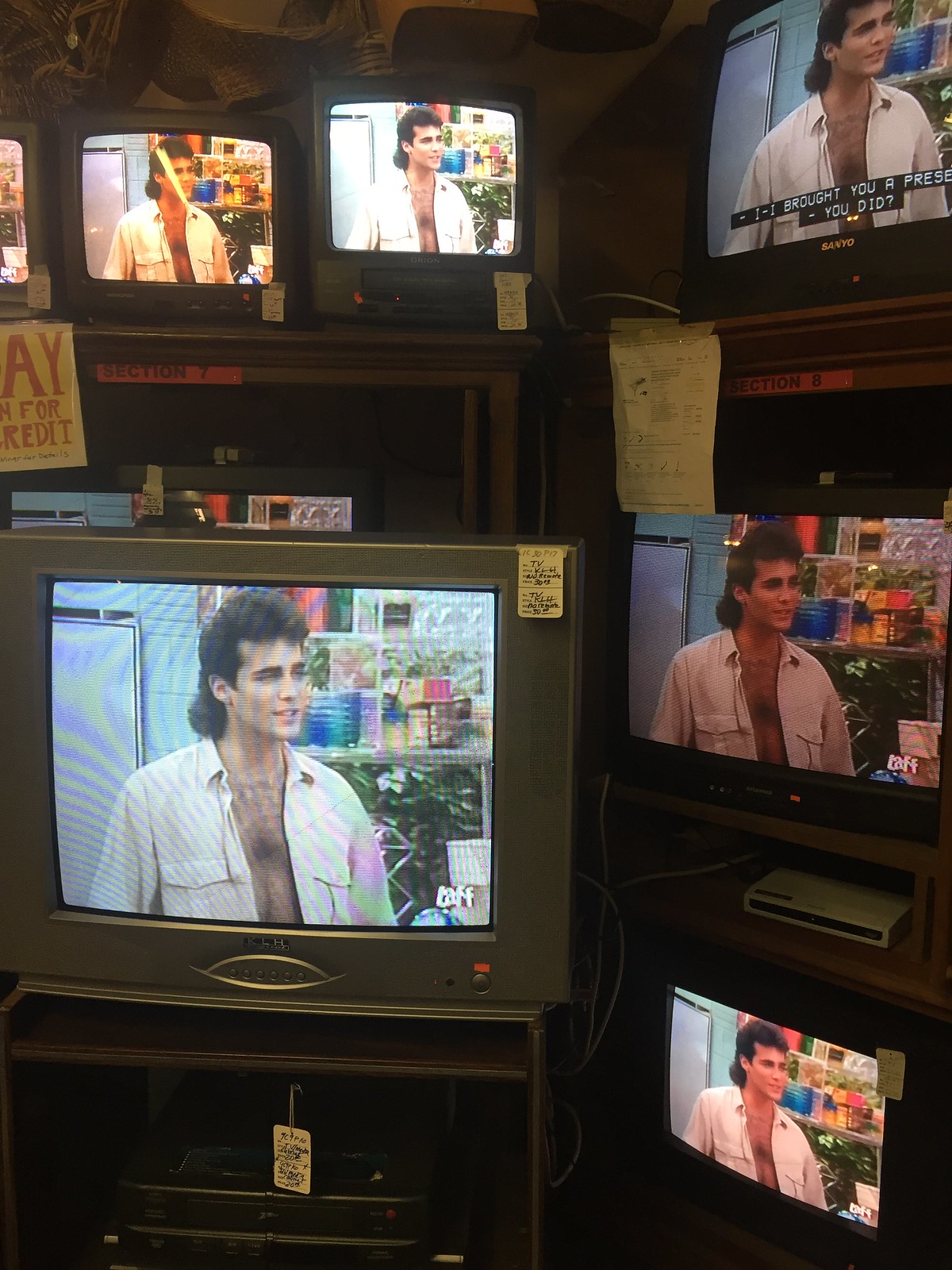In the photograph, an assortment of vintage CRT televisions is displayed in what seems to be a store setting, likely from the 70s or 80s due to both the models and the content shown on the screens. On the right, there are three televisions, one of which is a Sanyo, all tuned to the same show featuring a man with a brown mullet and an open-front, long-sleeved shirt, revealing a hairy chest and tan skin. This setup appears to have price tags or labels attached near the shelves. On the left side, there is a TV stand with three small TVs arranged closely together and one large silver-colored TV positioned in front of them. Additionally, VCRs are seen placed under and on top of some of the TVs, hinting at the older era of the display. All the televisions are showing an image of the same man, surrounded by flowers, reinforcing the nostalgic atmosphere of the scene.